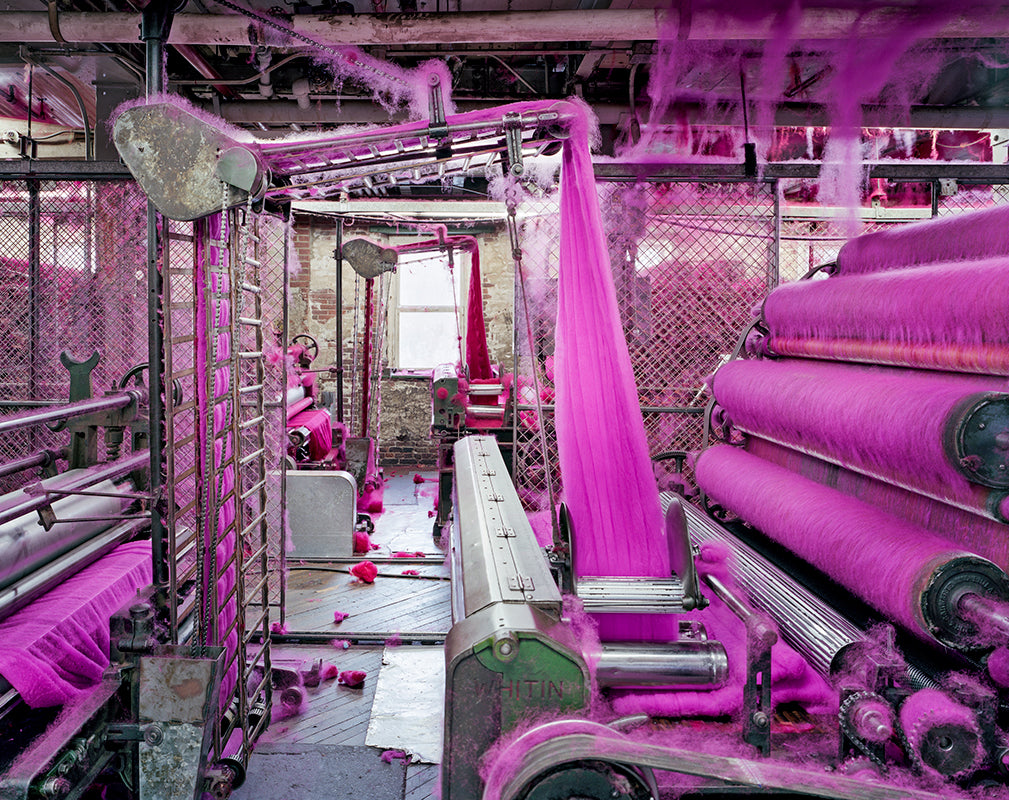This photograph, taken indoors at a commercial mill named Witten, showcases a disorganized and cluttered facility engaged in the production of bright pink fiber, possibly yarn, silk, or cotton. The scene is dominated by heavy machinery and rollers, primarily on the right side, which are enveloped in bright pink fibers. These fibers are spun and stretched across the center-right of the image before being funneled into a contraption above that aligns and processes them further. The output can be seen emerging on the left side of the image, suggesting the fibers are being transformed into thicker materials like blankets or towels. The room is encumbered with pink fibers intertwined with various equipment and hanging from the ceiling. The filthy white pipes and chain-link fences, all similarly encrusted with the pink material, contribute to the messy appearance. Notably, no persons are present in the photograph, and there are no additional identifying details as to the location of the facility beyond the "Witten" branding on the machine.